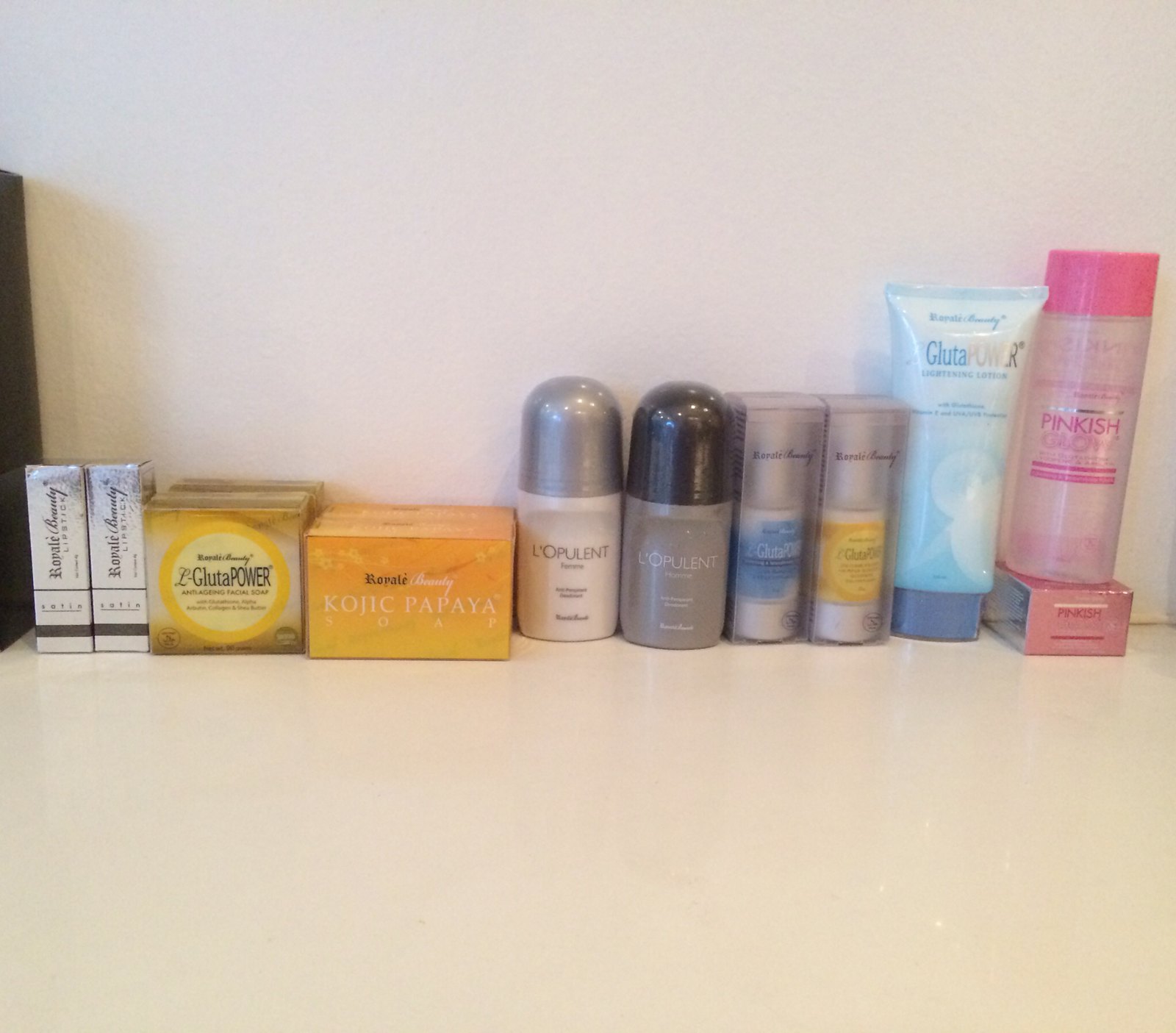In the photograph, taken in a minimalist bathroom, several BeautyAid products are neatly arranged in a single line on a smooth, white laminate countertop. The backdrop is a plain white drywall, which accentuates the array of products displayed. On the far left, there are two short, silver boxes marked with a logo that reads "something beauty," though the precise name is unclear. Adjacent to them is a square box branded with "something gluta power," featuring a gold circular design with shimmering accents. Following these are two boxes of kojic papaya soap, distinguished by their orangish labels. Next in line are two tubes of La Opulent—one with a light gray lid, the other with a dark gray lid, indicating variations of the product. Further to the right, two bottles with unreadable labels are seen, one adorned with a blue label and the other with a gold label. The lineup concludes with a blue squeeze bottle situated next to a pink liquid bottle, completing the collection of BeautyAid products on display.